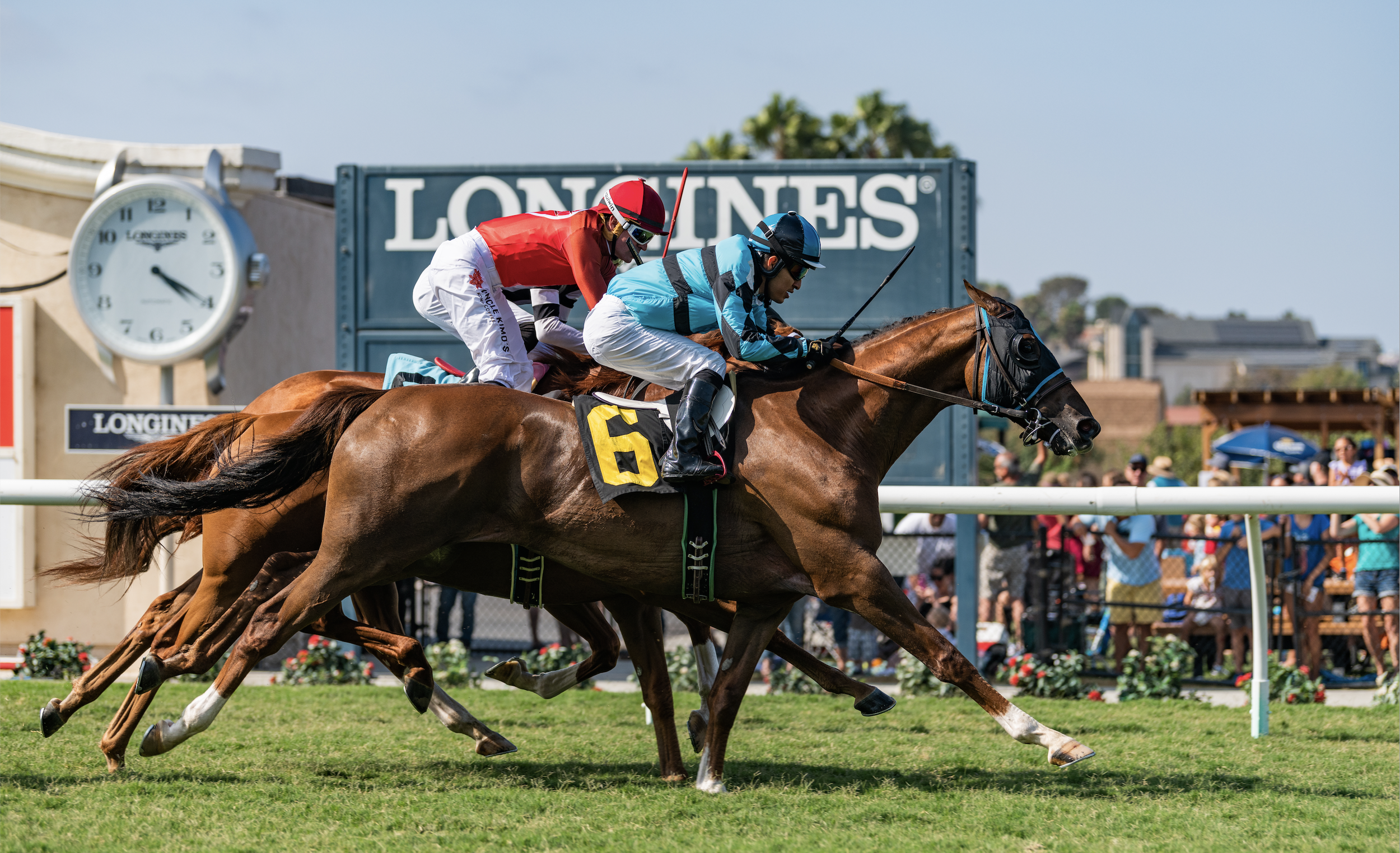The photograph vividly captures the intense moment of a horse race nearing its finish line under a pristine blue sky. Prominently featured in the foreground is a brown horse with a number six emblazoned on its black and yellow saddle blanket, ridden by a jockey clad in a light blue and black jersey, matching cap, and white pants. Close beside, another brown horse with a jockey dressed in solid red, with a red and black cap and white pants, races neck and neck. Although three horses are aligned, the third is partly obscured, revealing only the jockey's white pants. The race unfolds on a lush green grass field, bordered by a white railing. Just beyond the railing, an assembly of spectators watch eagerly, some sheltered under a blue umbrella. A large outdoor clock resembling a giant stopwatch indicates the time as approximately 4:20 PM. Adding to the scene's authenticity, a Longines scoreboard looms in the background, underscoring the event's formal sponsorship. Buildings are visible further to the right, providing a backdrop to this gripping race moment.